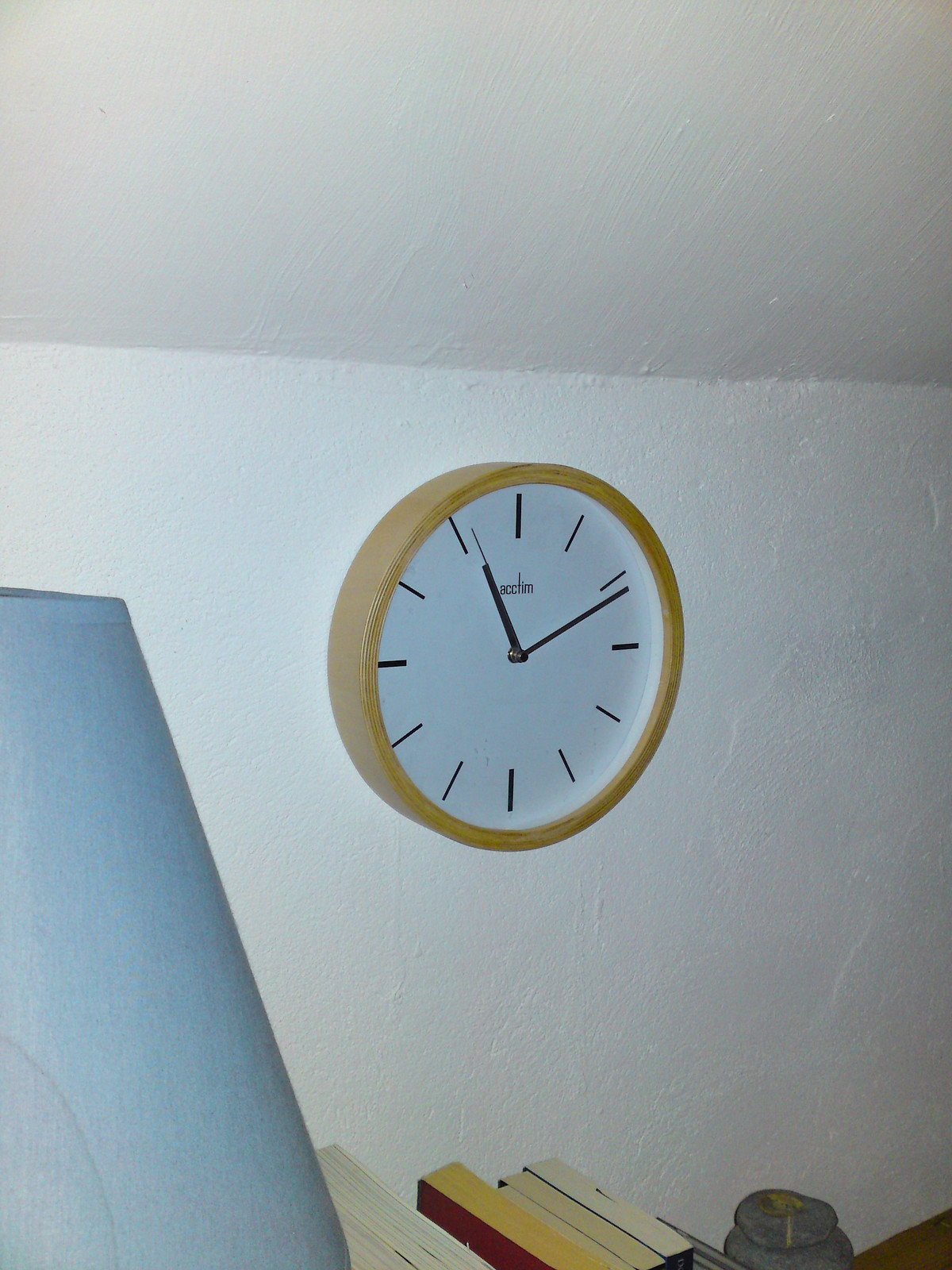This color photograph, taken inside possibly an attic or crawl space with a textured white wall and white ceiling, showcases a large, wooden circular-framed wall clock. The clock, set against the white backdrop, prominently features a plain white face with black hands and minimalistic black slashes instead of numbers, indicating a stopped time of 11:12. Below the 12 o'clock position, there's an illegible brand name. Adding to the room's simplicity, the lower left portion reveals a light blue object, likely part of a lampshade, while to the right, a shelf holds a stack of books showing their page edges. The floor beneath is red, completing the room's understated, utilitarian aesthetic.